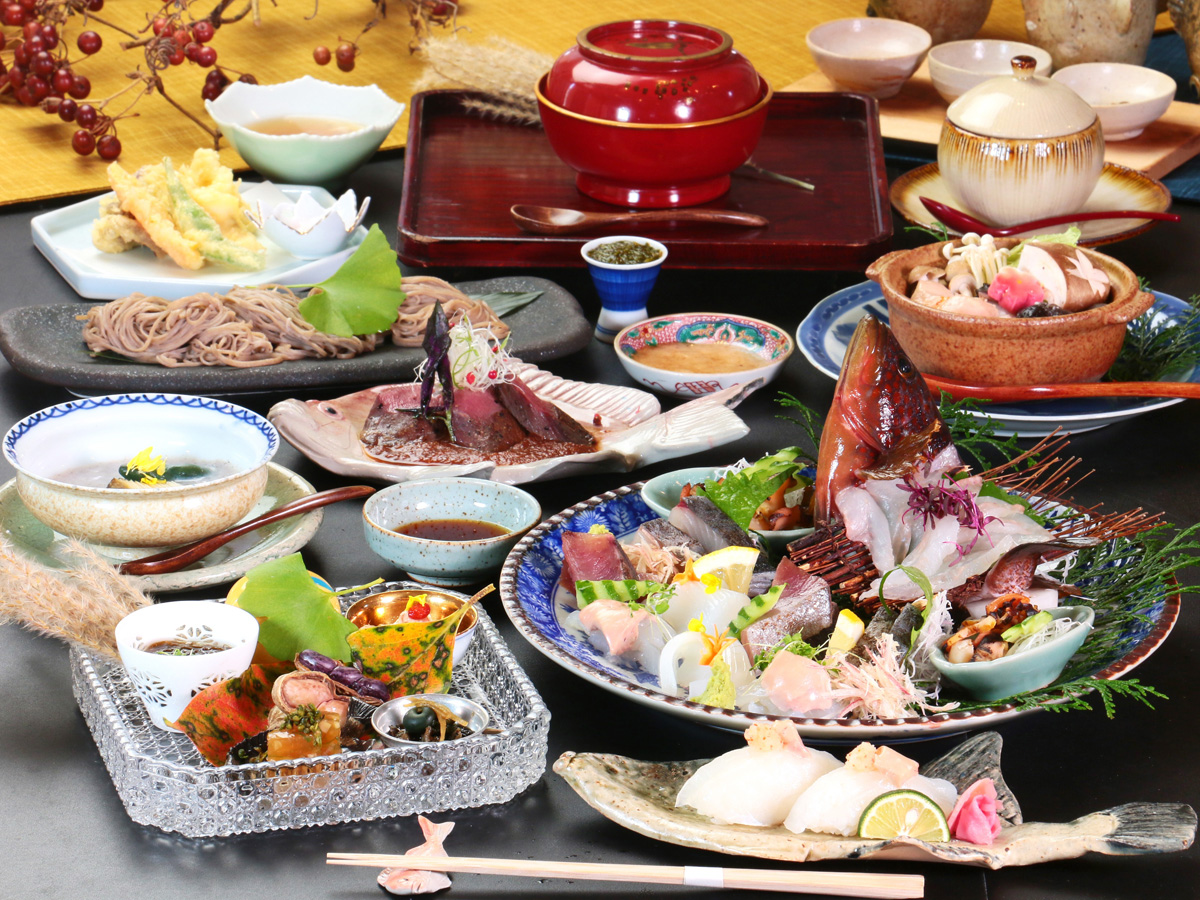The image showcases a diverse spread of dishes arranged on a black tabletop, primarily featuring various seafood items. In the foreground, chopsticks lie prominently, hinting at a setting suitable for Asian cuisine. Towards the bottom left, there's a clear square glass bowl adjacent to a blue bowl, while in the background on the left side, a series of smaller bowls lead up to a hexagonal bowl and a small white dish.

Centrally located is a distinctive fish-shaped platter adorned with pieces of fish and a lime, further surrounded by a mixture of other seafood offerings, including a brown fish head prominently sticking up from the plate. Adjacent to this is a salad bowl, and to its right, a brown bowl filled with pasta rests on a blue-patterned plate. Nearby, a beige and brown container with a lid and a red spoon stands out.

In the center back of the image, a dark cherry wood tray holds a large red bowl with a serving spoon beside it, and a couple of small bowls of sauce positioned in front. In the lower right quadrant, a blue plate supports a brown bowl, likely containing pasta or noodles, which is in proximity to another sauce bowl and a possible jar of unknown contents.

Towards the upper-left corner, the visual narrative completes with a cluster of red grapes and a series of small white bowls. The varied and colorful layout illustrates an intricately composed meal replete with foreign flavors and textures, alluding to a rich and diverse culinary experience.